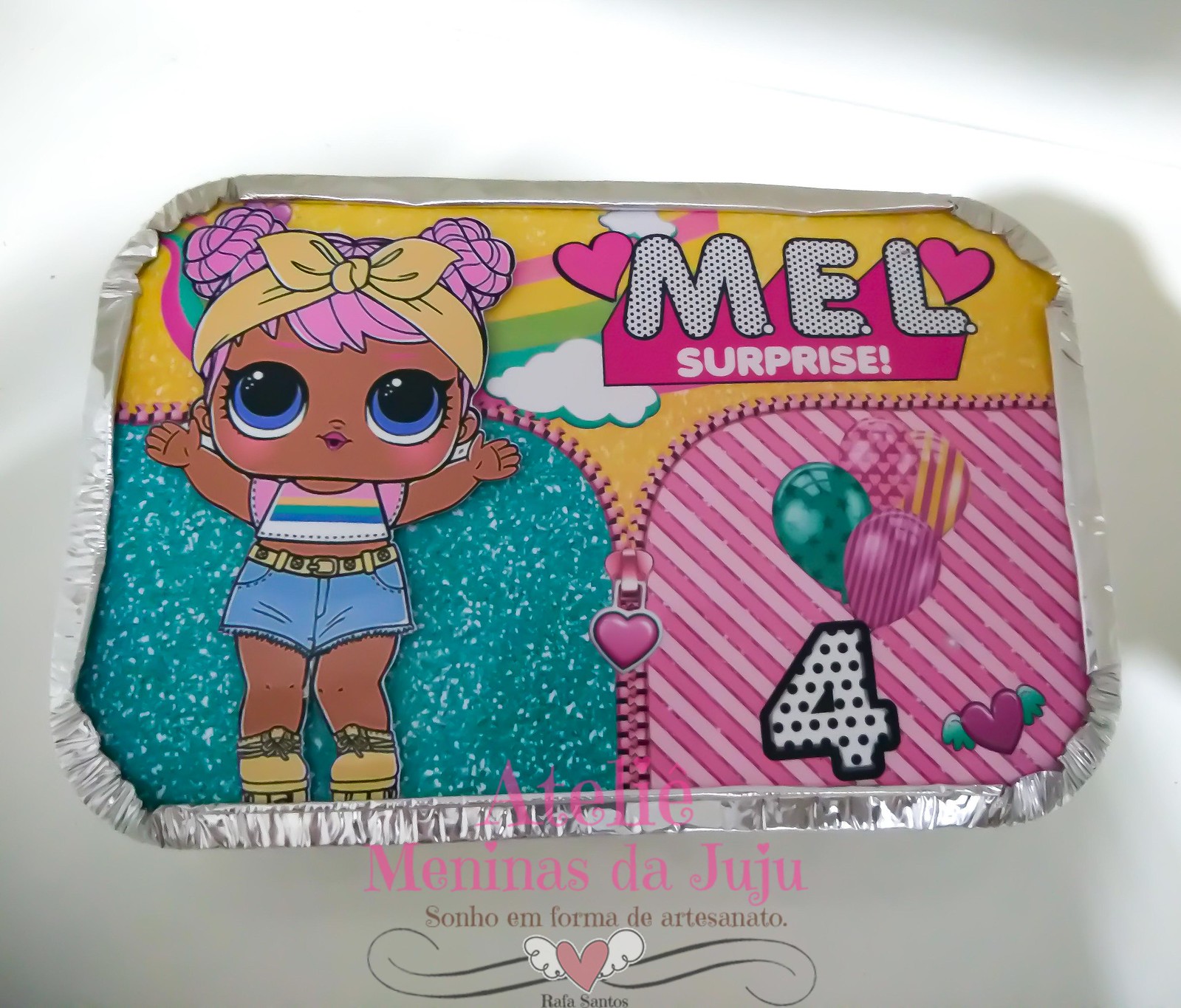The image features colorful packaging for a children's toy, prominently displayed on a white tabletop. The toy is encased in a silver tin foil container with an intricate, vibrant cover that exudes a playful, childlike aesthetic. The background includes a rainbow with clouds, and a color palette of pink, turquoise, white, and purple, among others. Centrally placed at the bottom, there is a watermark in another language, "Meninas de Juju," in pink letters, adorned with curvy lines and a pink heart with angel wings.

On the left side of the packaging, a charming illustration of a baby girl is featured. She has pink double bun hair tied with a yellow headband, blue eyes, blushing cheeks, a rainbow-colored t-shirt, denim shorts with a yellow belt, and matching yellow boots. To the upper right of this character, the text "M.E.L. Surprise" is displayed, surround by hearts and featuring a pink heart with white letters depicting "Surprise." A zipper motif runs through the middle of the design, with aqua-colored sparkles to the left and pink horizontal stripes to the right. The cover also includes a prominent black and white polka-dotted number 4 intermingled with balloons in blue, pink, and yellow colors. Additionally, there is a heart with wings in the bottom right-hand corner.

The overall setup and composition create a vivid and engaging visual, sure to catch the attention of children and stand out on store shelves.